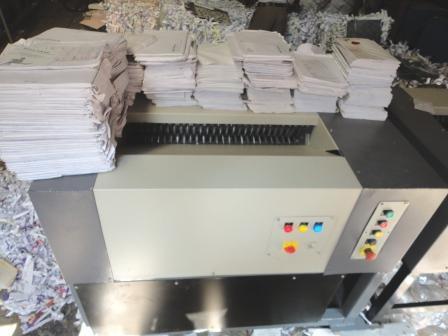The image showcases a commercial-grade shredding machine with a rectangular form, featuring an off-white/tan central section flanked by medium gray or silver sides. The front panel of the machine, shown at an angle, displays a series of buttons for operation. Three buttons—red, yellow, and blue—are aligned horizontally. Below them, there is another red mark set against a yellow background. To the side, on the right gray panel, there are five vertically aligned buttons in the sequence of green, red, yellow, black/gray, and red again. The top of the machine includes an opening section presumed to be the entry point for the papers. Stacks of paper, approximately seven to eight feet high, are organized on top of the machine, indicative of the machine's readiness to shred the papers. The background and the floor area around the machine are littered with shredded paper, reinforcing the machine's purpose as a shredder. The configuration and layout suggest this is a high-capacity shredder used in a commercial setting, rather than a household device.